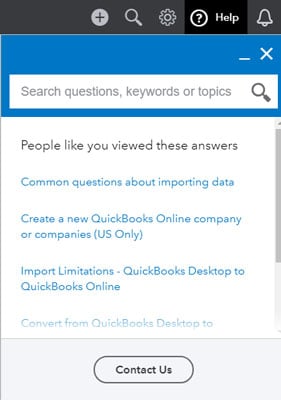This image is a screenshot of a cell phone displaying a help or support page. At the bottom center, there's a "Contact Us" button. Above this, there are three clickable links in blue font, each leading to different informational pages. The first link, at the top, reads "Common Questions About Importing Data." The second link, below it, states "Create a New QuickBooks Online Company or Companies, U.S.A. Only." The third link says "Import Limitations QuickBooks Desktop to QuickBooks Online." Above these links, a brief description indicates that other users have viewed these answers. At the top of the screen, there's a slim, rectangular search bar prompting users to "search questions, keywords, or topics," accompanied by a magnifying glass icon on its right. Further to the right are minimize and exit buttons for the screen.